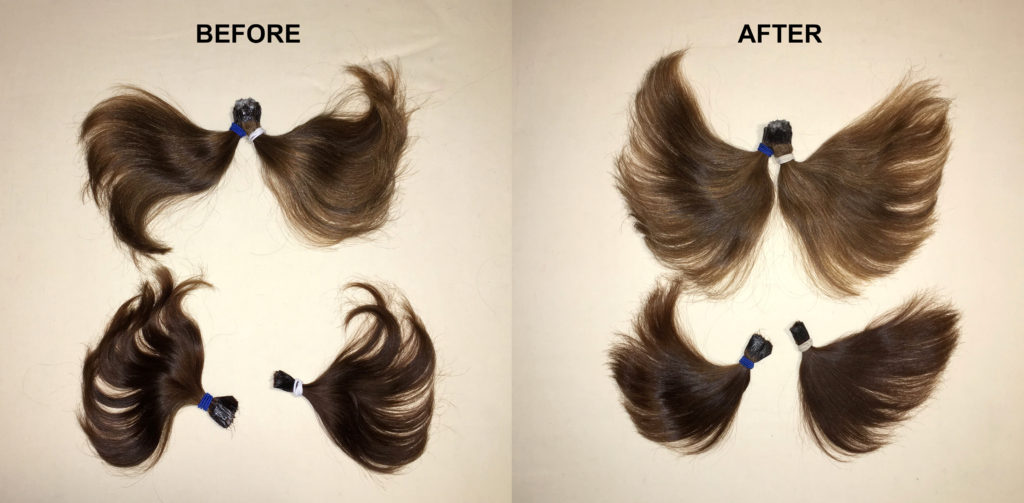The image consists of a side-by-side before and after comparison. The background on the "before" side is a light peachy color, while the "after" side features a mauve or purple hue. Both images are labeled at the top in black capital letters: "BEFORE" and "AFTER."

In the "before" picture, there are four clumps of hair tied tightly at the top with rubber bands. The two top clumps are close together, touching slightly and resembling wings, while the ones at the bottom are more separated and appear less organized.

Contrastingly, the "after" picture shows a significant difference. The top clumps remain close together in a wing-like formation but are combed very neatly, looking soft and well-groomed. The bottom clumps, although not touching, also present a neat and clean appearance, showcasing a considerable improvement in tidiness compared to the "before" side. The overall clarity of the images is excellent, with a bright and well-lit setting.